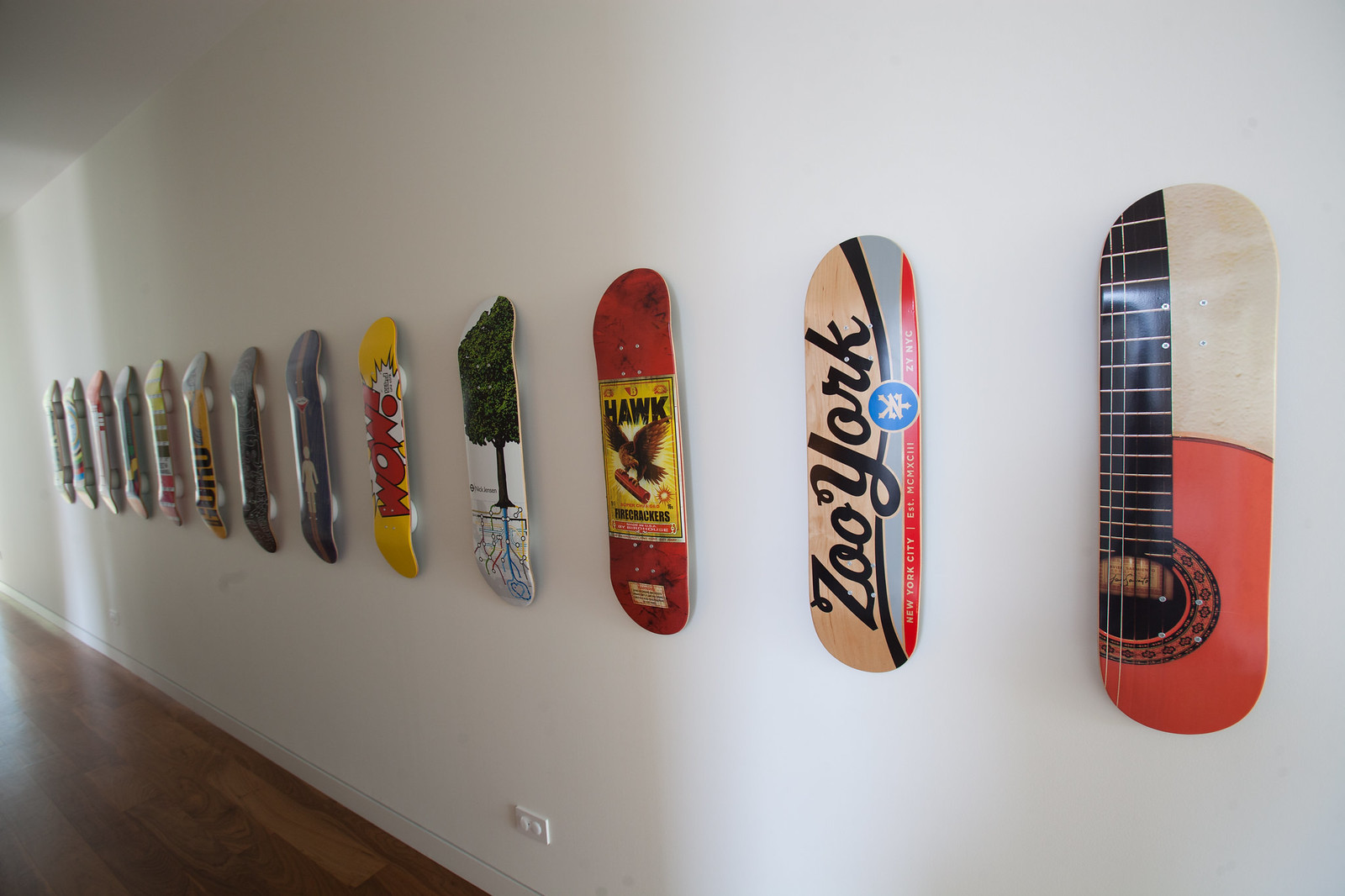An angled image captures a bright, white-walled room featuring a stylish and artistic display of 13 skateboards mounted in a row. Each skateboard is different, showcasing a variety of vivid designs that are mounted without wheels, appearing almost like art pieces. As the eye moves from left to right, the skateboards come into sharper focus. On the left, the boards are partially out of focus, while in the middle, a vibrant yellow board with a pop art style exclaims "WOW" in bold comic book font. To the right, another skateboard features a striking design of red, white, and black, with the word "New York" in black text. Behind some boards on the left, you can see they're held by two white discs. The room's clean aesthetic is enhanced by a shiny, wooden parquet floor visible in the bottom left corner and a discreet electric socket. The diverse and eclectic skateboard designs create a visually stimulating and stylish display, giving the impression of a curated art installation.